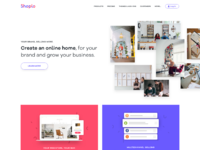The image depicts an extremely blurry web page, which seems to be for a site named "Shanjin." In the upper left-hand corner, there is text in pink and blue colors. To the right of this text, a horizontal menu bar features five menu options in black, though the specific text is illegible. Located in the upper right corner is a blue and white oval-shaped button, the text on which is also unreadable.

Central to the page, some legible black text reads, "Create an online home for your brand and grow your business." Below this statement, there is an oval-shaped button with blue text that cannot be made out due to the blur. On the right side of the page, six photographs are arranged in a circular overlapping pattern. 

At the bottom, the page features two boxes: a pink one on the left and a blue one on the right, though their contents are indiscernible.